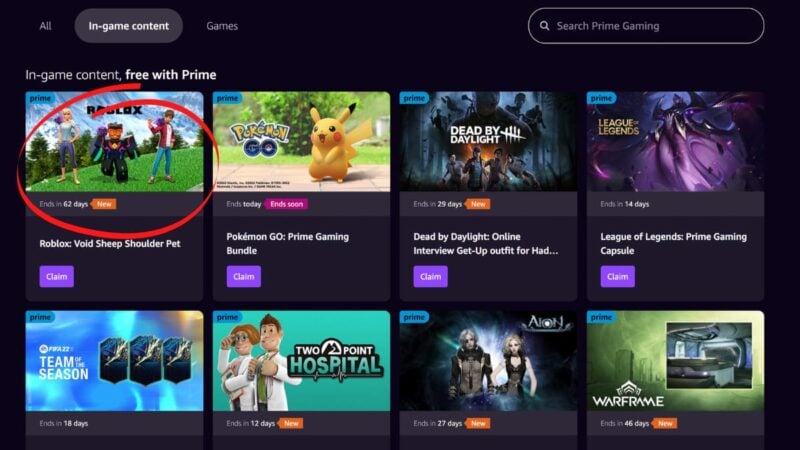The screenshot showcases the Prime Gaming website, set against a sleek black background. The webpage features two horizontal rows, each consisting of four distinct sections displaying various offerings. At the top, the header reads, "All in-game content, games," accompanied by a search bar on the right side, labeled, "Search Prime Gaming for in-game content, free with Prime." 

The upper row prominently displays images of available games and their associated content:
1. **Roblox** - highlighted with a red circle, showcasing the "Void Sheep Shoulder Pet."
2. **Pokemon Go** - featuring the "Prime Gaming Bundle."
3. **Dead by Daylight** - spotlighting the "Get Up Outfit for MAD."
4. **League of Legends** - presenting the "Prime Gaming Capsule."

The bottom row offers additional selections of in-game content:
1. **FIFA Team of the Season** - a notable sports game feature.
2. **Two Point Hospital** - offering an undisclosed in-game item or bonus.
3. **Aion** (stylized as A-I-O-N) - presenting a mysterious in-game content.
4. **Warframe** - featuring yet another exclusive item or offer for players.

Each game’s section is visually represented with engaging images that entice users to explore the exclusive in-game content available through Prime Gaming.